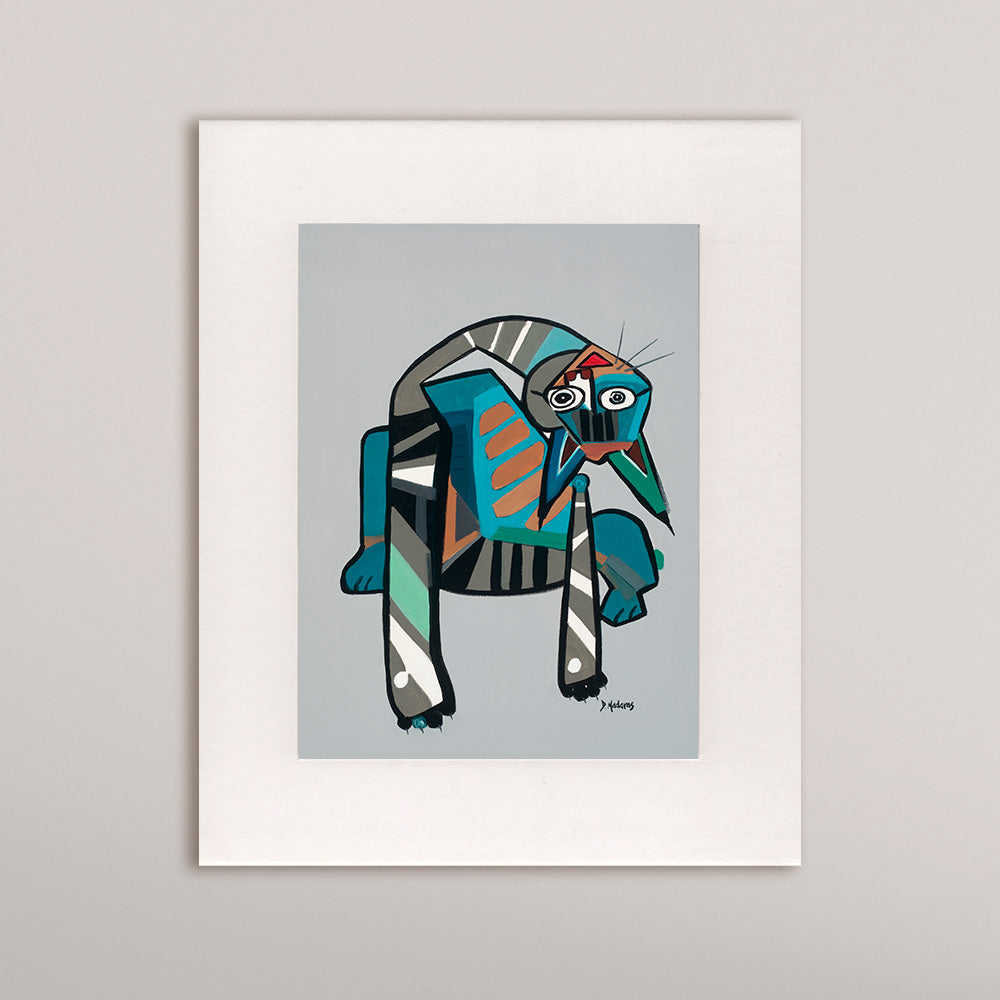This photograph captures an eclectic and abstract piece of artwork, evocative of modernist styles like that of Pablo Picasso. The artwork is displayed on a white mat within a tall, rectangular frame, set against a very light gray wall, possibly suggesting that it is hung for sale or display. The image depicts a cat in a highly stylized manner, featuring a skewed and asymmetrical anatomy. The cat has vibrant, diverse colors, predominantly shades of gray and teal, with added accents including orange stripes on its belly, an orange chin, and a bright red mouth. The cat's legs are teal green, while its long, giraffe-like neck twists to position the head upside down, making the ears point downward—one ear green and the other blue. The face is engaging with two eyes directly gazing out and whiskers solely on the right side. The legs and arms have muted claw-like structures with patterns in gray, white, black, and green. The artwork bears a small, somewhat illegible signature at the bottom right corner, which seems to read "D. Medaros."